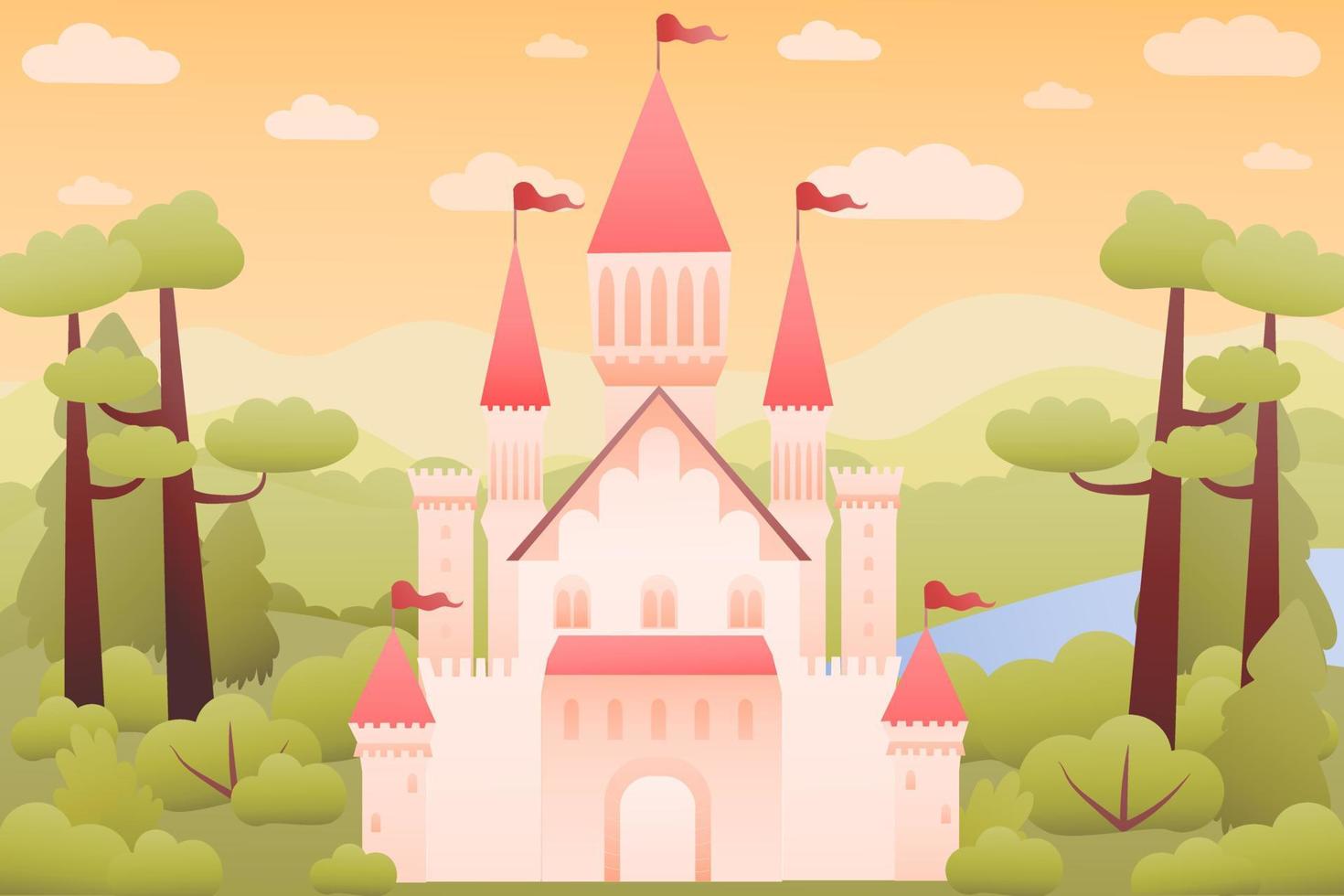This digitally drawn image showcases a cartoony, vectorized illustration of a picturesque pink castle, prominently centered in a lush, forested landscape. The castle, reminiscent of a Disney princess castle, features a light pink exterior with multiple conical towers topped with deeper pink, gradient-shaded domes. Each of the five pointed spires has a red flag billowing to the right. The castle is surrounded by tall, simply drawn green trees and bushes with varying shades of green, adding a whimsical touch to the scene. The background reveals a serene river and distant mountains under an orange-yellow sky adorned with fluffy white clouds, enhancing the enchanting, fairy-tale ambiance of the image. The entire composition is rendered in a simplistic, mobile game-style art, emphasizing the charming and playful nature of this castle in a forest setting.